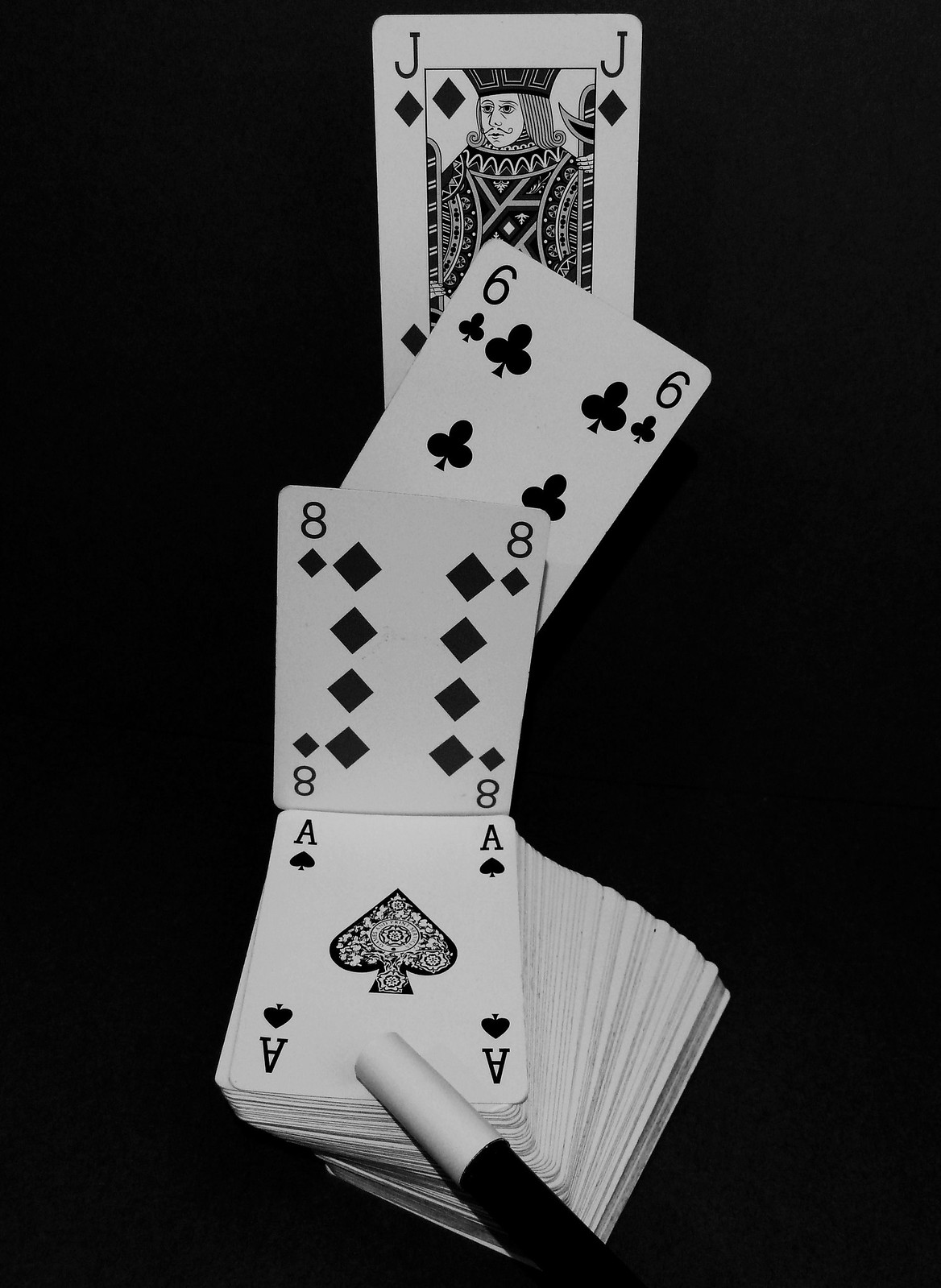In this striking black and white photograph set against a dark background, a deck of playing cards takes center stage. The cards, notably the Jack of Diamonds, Six of Clubs, Eight of Diamonds, and the Ace of Spades, are beautifully arranged with the latter card prominently displayed. The cards are slightly fanned out beneath the Ace of Spades, creating a layered effect. Adding to the magical ambiance, a classic magician's wand with white tips rests delicately on the Ace of Spades, suggesting an air of mystery and enchantment. The monochromatic palette enhances the dramatic and timeless quality of the scene.